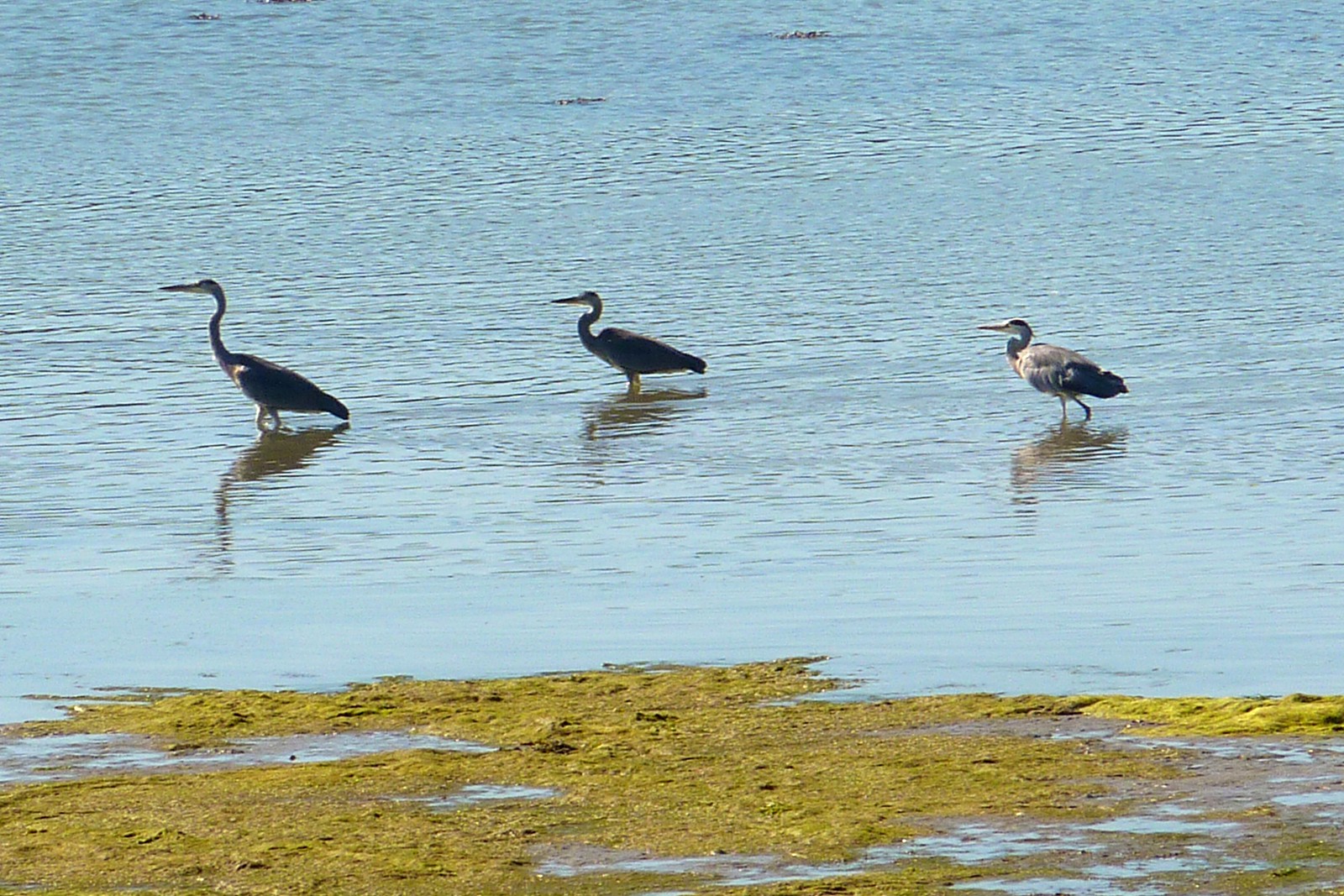This is a tranquil wildlife nature photograph capturing three birds standing in shallow, calm blue water. The scene is peaceful, with no wind or waves disturbing the surface. The foremost part of the image features a greenish-brown moss, suggestive of swamp or shallow water conditions, which indicates the varying depths of the water. The three birds, likely a type of long-legged waterfowl like herons, egrets, or a similar species, are positioned in a line, all facing the left. The bird on the far left is the largest, black with a long neck. The middle bird, similar in appearance but smaller, also has a black long neck. The bird on the right is the smallest, with a more compact build and distinctive coloring: white body feathers and black feathers on its head, back, and tail. Their feet are submerged, suggesting a very shallow area, and their differing sizes and positions add depth and interest to the serene setting.